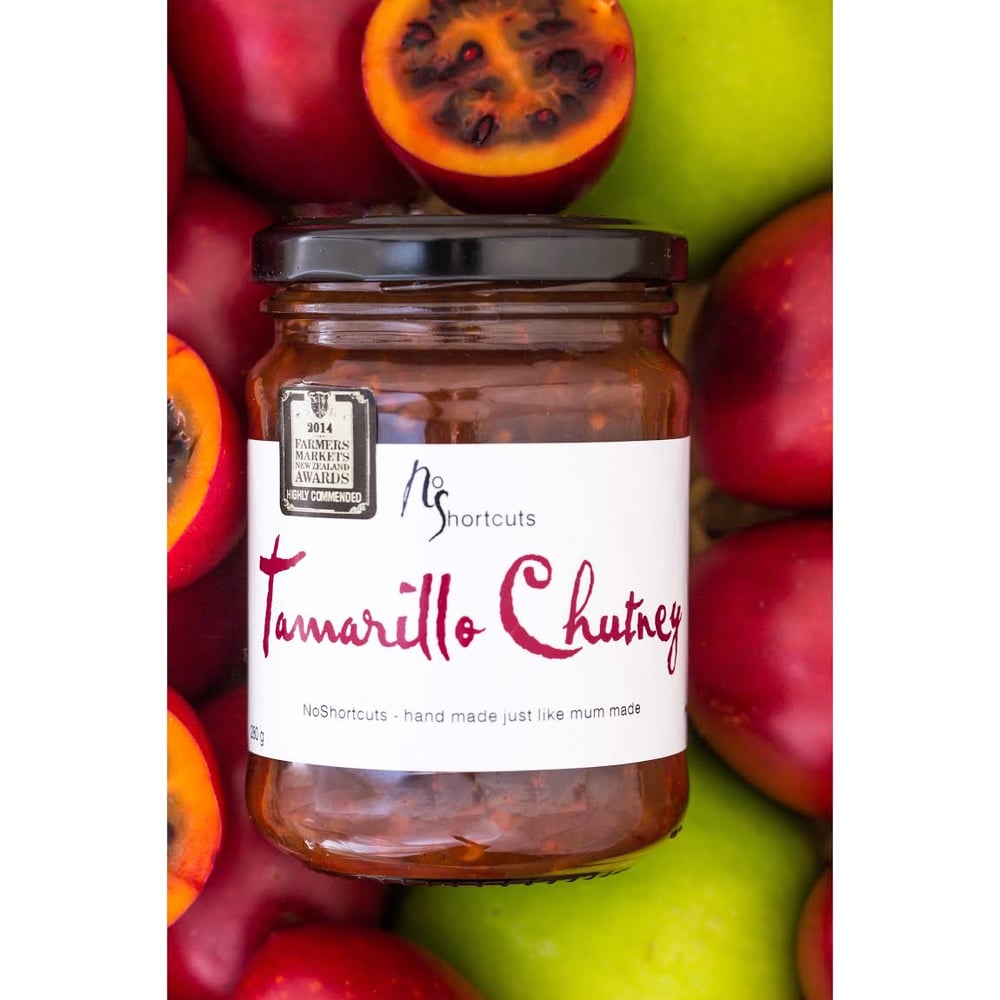In the center of the photograph is a clear glass jar with a black metal screw-on lid. The jar is filled with a red substance, identified as Tamarillo chutney. A white label on the jar is detailed with black text reading "no shortcuts" at the top, followed by "Tamarillo chutney" in large red script in the center, and "no shortcuts, handmade just like mom made" in smaller black text at the bottom. In the upper left corner of the label, there is a black and beige sticker that reads "2014 Farmers Markets Award, highly commended." The jar is surrounded by an assortment of fruits, primarily red and green in color. Some of the fruits are whole, while others are cut in half, revealing a vibrant orange interior with small seeds. These fruits appear to be tamarillos, contributing to the thematic context of the jar's contents.